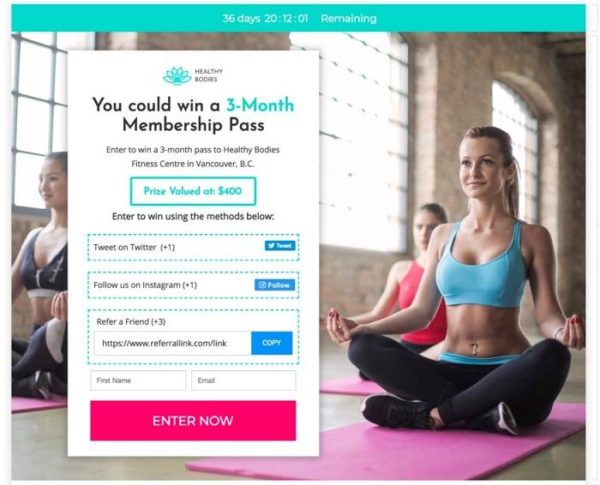The image depicts a promotional webpage for the "Healthy Bodies" fitness center. The header, set against a teal-blue background, displays a countdown timer with the numbers "36 days, 20:12:01 remaining" in white text, indicating the time left to enter the promotion. The main background features an image of women practicing yoga, seated cross-legged with their palms resting on their knees in a meditation pose. The most prominently visible woman has blonde hair, light skin, and is dressed in a blue sports bra and leggings.

On the left side of the webpage, a sign-up section is titled "Healthy Bodies," accompanied by a flower logo. The heading advertises a chance to win a "three-month membership pass," with "three-month" highlighted in light blue. Beneath this, a description invites users to "enter to win a three-month pass to Healthy Bodies Fitness Center in Vancouver, BC," stating the prize valued at $400 in a blue outline. The section includes several ways to enter: tweeting on Twitter, following on Instagram, and referring friends for additional entries (+3, +6).

Further down, fields for "First Name" and "Email" prompt users to input their information. The sign-up form concludes with a prominent pink-purple button labeled "Enter Now."